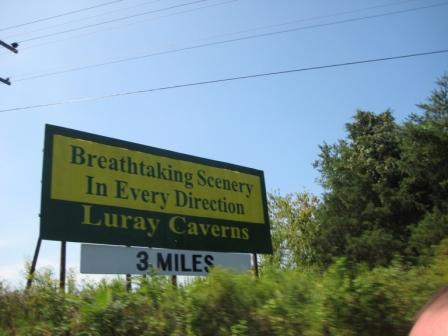This daytime photograph features a vivid blue sky accentuated by black power lines stretching across the upper portion of the composition. Below the power lines, a prominent billboard captures attention with its striking black and yellow design. The billboard, against a black background, displays a yellow rectangle with bold black text that reads, "Breathtaking scenery in every direction." Below this, in bright yellow font, the name "LURAY Caverns" stands out, followed by a white rectangle with black text indicating, "3 miles."

Flanking the billboard, dense green trees span the spectrum from deep forest green to lighter shades, adding a lush natural border to the scene. At the bottom of the image, overgrown shrubbery in various hues of dark green, yellow-green, and light green adds texture and depth. The image quality is commendable, with only a slight blur that does not detract from the overall clarity and detail of the scene.